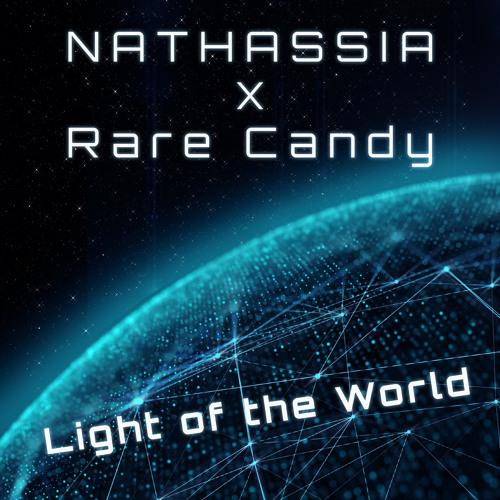This computer-illustrated poster features a captivating, dark night sky as the background, dotted with sparkling stars suggesting a distant galaxy. Dominating the lower half is a striking half-globe rendered in green hues reminiscent of the Matrix, crisscrossed with glowing green lines and punctuated by bright green dots. This globe evokes a digital or technological theme, blending monochrome blue and black, creating a futuristic aesthetic. In the upper part of the poster, the name "Nathassia" is prominently displayed in white font, followed by an "X", and then "Rare Candy" below it, all elegantly aligned. The lower half is emblazoned with the phrase "Light of the World" in white font, slightly tilted upwards, resonating with the illuminated grid of the globe below.